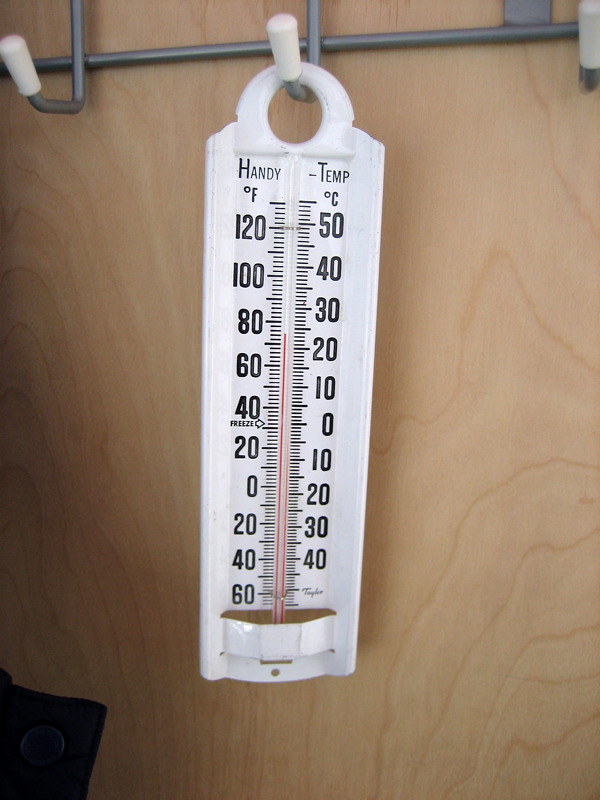The image features a temperature thermometer hanging from a silver hook with a small white knob. This thermometer is primarily white, with temperature readings marked in bold black numbers. A red mercury line indicates the current temperature. The thermometer, branded with "Handy Temp" at the top, displays both Fahrenheit and Centigrade scales: the Fahrenheit scale ranges from -60 to 120 degrees, while the Centigrade scale ranges from -40 to 50 degrees. The thermometer is suspended against a beige wooden wall, creating a simple backdrop. The current reading is approximately 75 degrees Fahrenheit. Overall, the image's color palette includes white, black, red, beige, and silver.